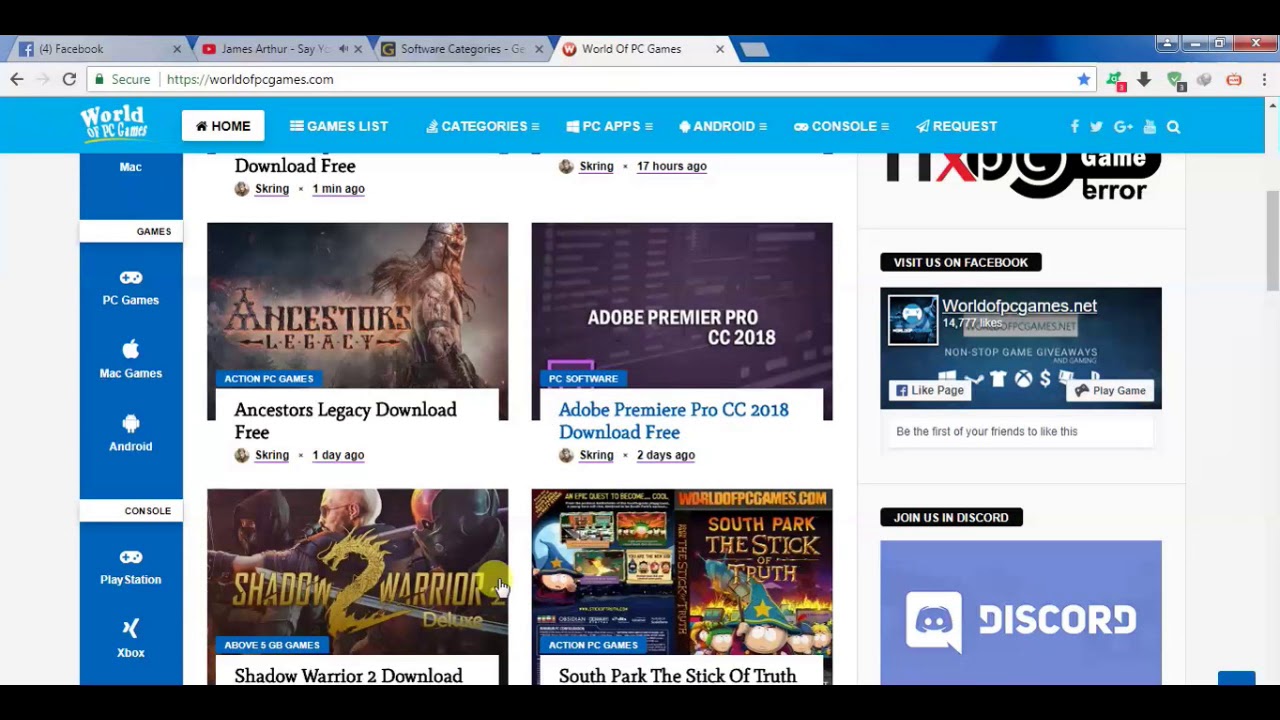The image showcases a computer screen with multiple browser tabs open. The screen features a black bar at both the top and bottom. The first tab displays Facebook, followed by YouTube opened to a James Arthur video. The third tab is a software category website, and the fourth tab opens to the World of PC Games website.

The World of PC Games page has a detailed menu bar that includes options such as Home, Games List, Categories, PC Apps, Android, Console, and Requests. Additionally, the page displays several social media icons for Facebook, Twitter, Google, an unidentified icon, and a search tab.

The current open section of the World of PC Games website features a selection of downloadable games and software, including Ancestors Legacy, Adobe Premiere Pro CC 2018, Shadow Warriors 2 Deluxe, and South Park: The Stick of Truth. Each game listing shows a thumbnail image, the sharer's name, and the number of days since it was shared. On the left side of the website, there is additional information likely intended to help refine searches. On the right side, there are tabs for accessing the Discord channel and the worldpcgames.net website.